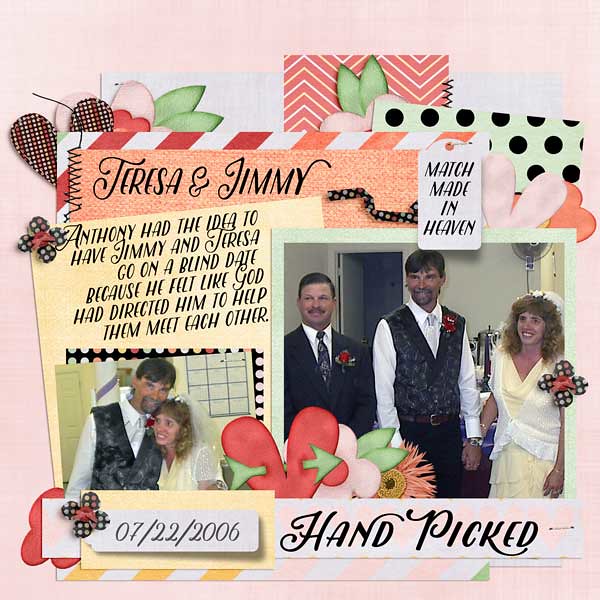In the center of this wedding photo collage, the groom stands proudly in a gray and black vest, black pants, and a black tie, with a red flower pinned to his left lapel. To his left, the bride, adorned in a pristine white dress with a big bow on her lapel, displays her long brown hair and radiates happiness as they hold hands. The father of the bride or groom, dressed in a dark suit, stands to the lower right wearing a matching boutonniere. The pink background at the top displays "Teresa and Jimmy" in an elegant script, with captions in rectangular sections detailing their love story. On the left, it explains that Anthony believed God directed him to set them up on a blind date. On the right, the sentiment "Match Made in Heaven" is enclosed in another rectangle. Below their primary portrait is a smaller photo of the bride and groom embracing, their foreheads touching affectionately. Beneath this image, encapsulated in a white rectangle, is their wedding date: 7-22-2006. Romantic elements, including hearts and butterflies, adorn the surrounding scenery, completing this touching depiction of love and fate.